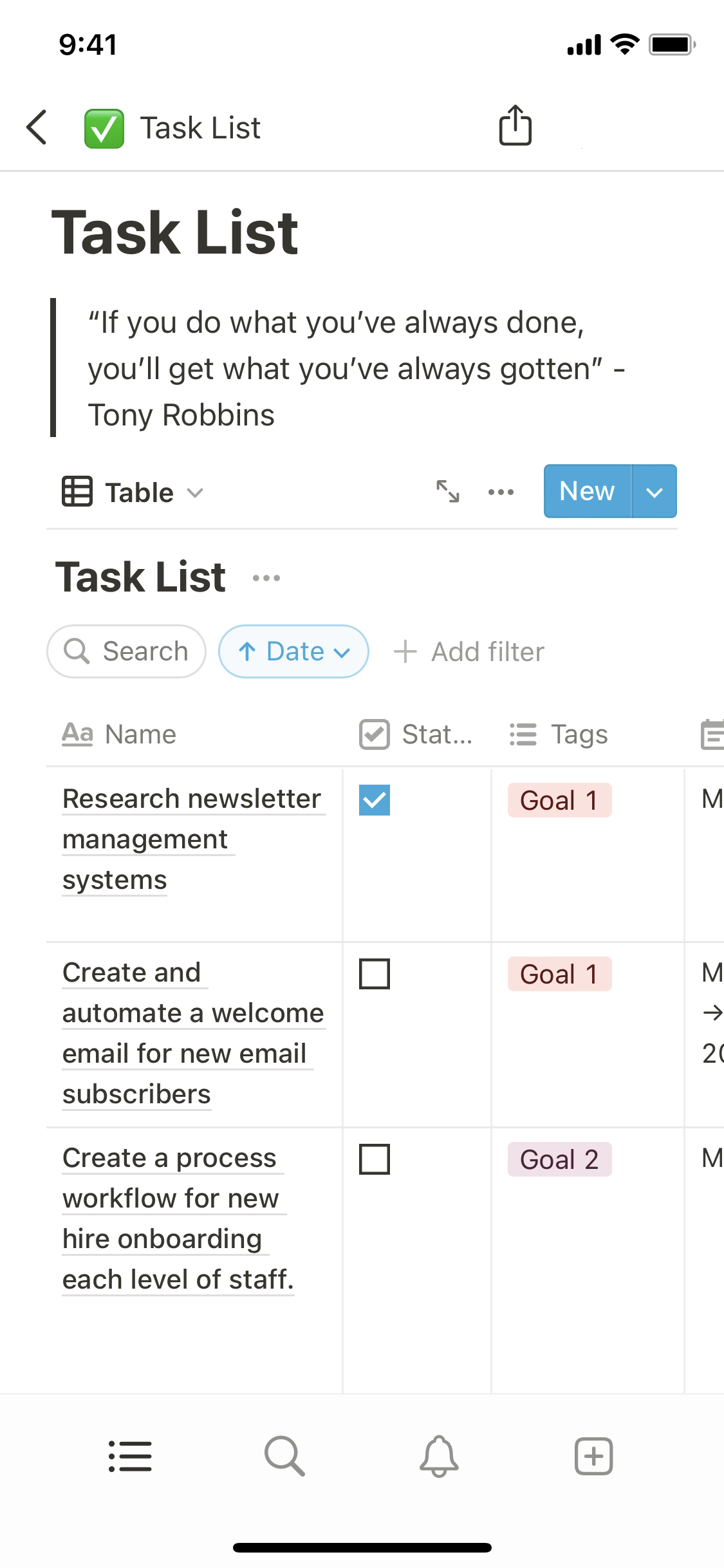The image depicts a screenshot of a task management app displayed on a smartphone. The interface shows a white background in the header area at the top, where the time is displayed as 9:41 AM on the left. The battery level, Wi-Fi signal, and cellular signal icons are visible on the right.

Below the header, there is a back arrow icon on the left, followed by a green square with a white check mark inside it. Next to the square is text that reads "Task List" in black font. Directly below, there is a larger text section in bold that also reads "Task List."

The following line features a motivational quote attributed to Tony Robbins: "If you do what you've always done, you'll get what you've always gotten."

The next section includes a table with a drop-down menu, indicated by a small arrow pointing downwards. To the right of this section, there are three vertical dots that commonly signify additional settings or options.

Further down, there is another drop-down menu with a blue background and white text. An additional line goes across the screen, followed by another "Task List" label adjacent to three vertical dots. 

The search bar is located below this, followed by a specific date in blue and an arrow indicating another drop-down menu. Next to this, there's a "plus" icon labeled "Add Filter."

The main body of the interface lists various tasks with different categories, including:
- Name
- Status
- Tags
- Research newsletter management systems
- Create and automate a new welcome email for new email subscribers
- Create a process workflow for new hire onboarding for each level of staff.

The structured and detailed layout seems designed to facilitate efficient task management and tracking.